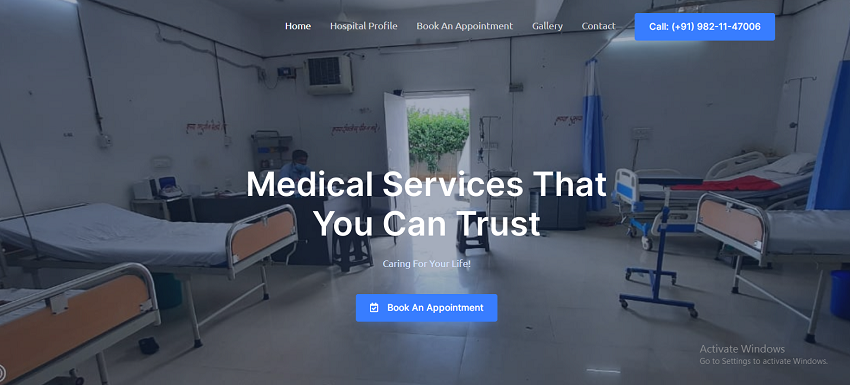Screenshot of a comprehensive medical services website. The background is muted, emphasizing the core message rather than visual details. Prominently displayed is a headline in bold, reassuring font: "Medical Services That You Can Trust." Below, a subheading reads: "Caring for Your Life." A clear call-to-action button labeled "Book an Appointment" is prominently situated, facilitating online bookings.

In the top corner, a conspicuous blue rectangle contains the word "Call" followed by a phone number, encouraging immediate contact. The navigation bar at the top of the page includes options such as "Home," "Hospital Profile," "Book an Appointment," "Gallery," and "Contact," enabling easy maneuverability through the site.

The background photo features a well-kept hospital room, equipped with several hospital beds, giving viewers a glimpse into the professional medical environment. An open door and a desk occupied by a healthcare provider further depict the active, caring nature of the services offered. The layout and design accentuate the user-friendly and approachable ethos of the medical website.